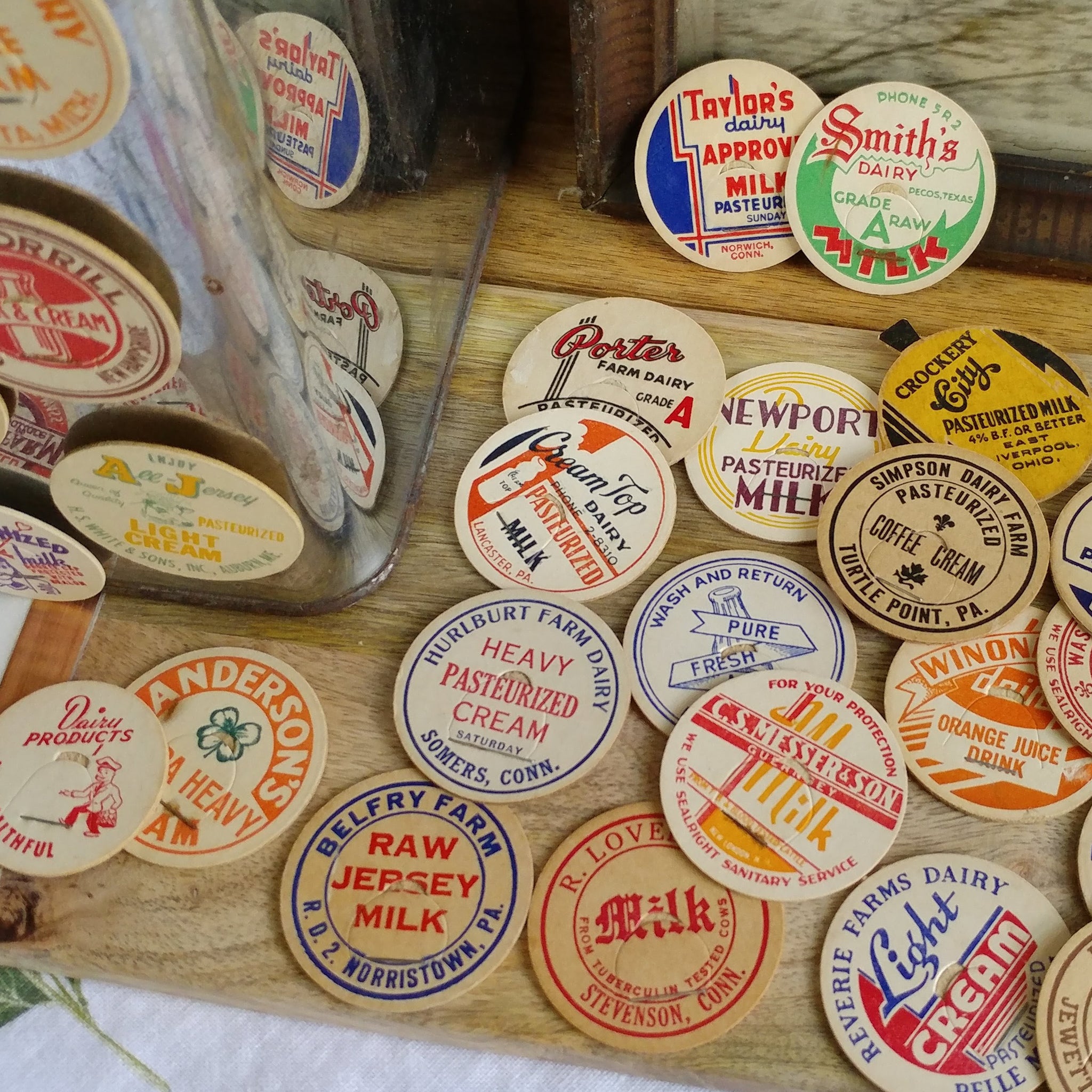This photograph features a diverse assortment of circular tokens, likely made from wood or cardboard, displaying advertisements from various dairy farms. The tokens, which are scattered across a wooden surface—possibly a table or floor—range in color and style, featuring red, blue, yellow, purple, orange, and green text. Each token includes distinct details, such as the names and products of different dairies. 

Prominent examples include Belfry Farm Raw Jersey Milk from Norristown, PA, Hurlburt Farm Dairy Heavy Pasteurized Cream from Summers, Connecticut, and Smith's Dairy Raw Milk. The tokens generally have the dairy name curved at the top and location information curved at the bottom, with product descriptions in the center. Some are even stuck to a metal object, suggesting they might be magnets. Though mostly advertising dairy products like milk and cream, there's even a mention of an orange juice drink, adding variety to the collection. The tokens appear to be about the size of a large coin, slightly bigger than an old-fashioned silver dollar.